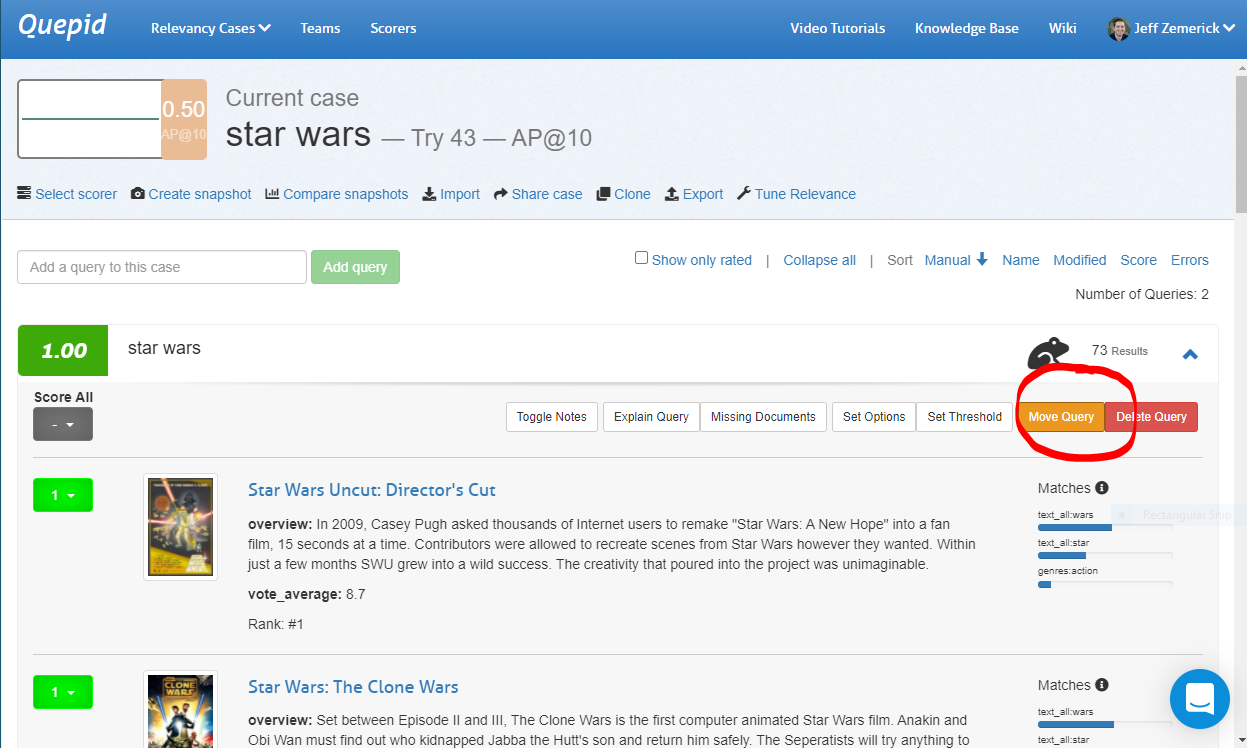The image is a screenshot from a website named QPID, uniquely spelled as Q-U-E-P-I-D, viewable in the top left corner of the page. In the top right corner, there is a user profile displaying the name and picture of Jeff Zimerick, who appears to be a Caucasian male.

The central section of the webpage highlights two movies: "Star Wars Uncut Director's Cut" and "Star Wars: The Clone Wars." Each movie listing features different rankings, average ratings, and detailed summaries providing insights into the films.

On the right side, several buttons are present, but one in particular stands out due to a red circle around it. This highlighted button is orange and titled "Moo Curry." 

Additionally, in the bottom right-hand corner, there is a chat option signified by a small white message bubble adorned with a smiley face at its base.